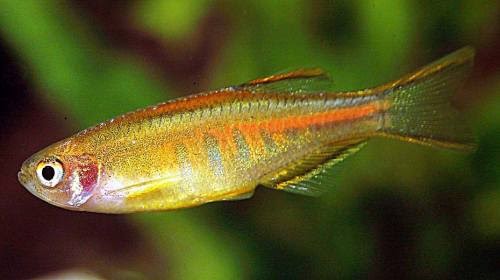The image features an up-close, highly detailed photograph of a small fish, likely a guppy or a similar beginner aquarium species. The fish, primarily greenish-yellow with golden accents, is adorned with orange lines along its back and belly, and soft pink blushing near its gills. Its eyes, which occupy most of its face, are iridescent and silvery with dark pupils. The tail and the back half of its fins are almost transparent with a glimmery texture, exhibiting shades of yellow and green lined with gold. The fish, appearing very tiny, possibly an inch and a half in length, is centered against a backdrop of blurry green foliage, likely from an aquarium plant, giving the impression of it floating in mid-water. The overall color composition of the image includes muted greens, browns, and blacks in the background, enhancing the shimmering, almost sparkly appearance of the fish.